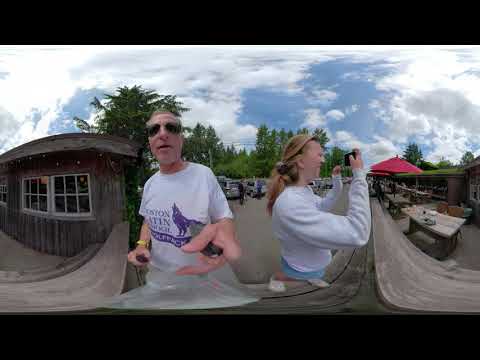In this outdoor photograph, taken with a fisheye lens or in panorama mode resulting in some distortion, we see two older Caucasian individuals against the backdrop of what appears to be a tourist location with restaurants and parking. 

In the foreground, on the left, is a man in his 50s with short, white hair and wearing sunglasses. He sports a white t-shirt featuring a blue design of a wolf howling at the moon and some unreadable text. He is holding a selfie stick to take the photo. 

To his right stands a woman, also in her 50s, with reddish-blonde hair tied back in a ponytail. She is dressed in a long-sleeved white sweatshirt and blue pants, and holds up a cell phone as she looks off to the right.

Behind them, there are rows of parked cars in a lot, tall pine trees, and houses. To their left, part of a wooden shack with white grid windows is visible, and to their right, one can see wooden picnic tables and benches under red umbrellas, suggesting a dining area. The sky above is partly cloudy with patches of blue, indicating a bright and pleasant day. The image's distortion notably elongates and flattens some body features, particularly affecting the woman’s face and limbs.